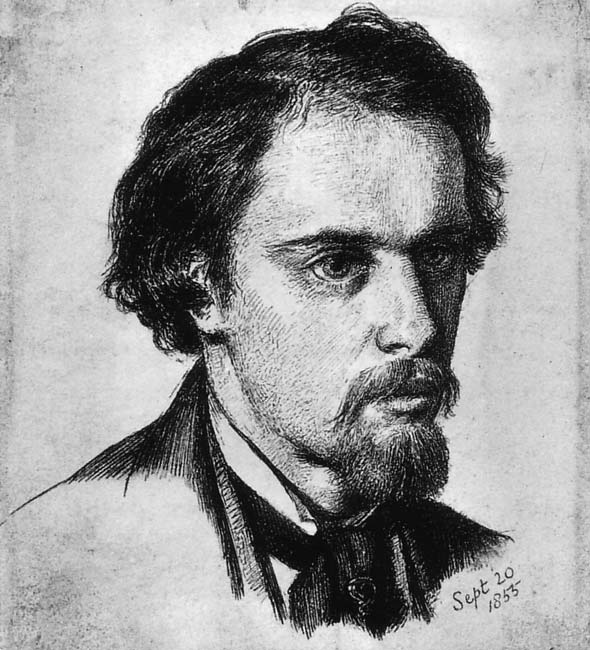This black-and-white sketch, executed with pencil or charcoal, is a self-portrait titled "Self-Portrait of the Artist 683" by Dante Gabriele Rossetti, created on September 20, 1855. The artwork captures an older man, approximately 35-40 years old, with dark hair neatly parted and combed to the side. He has sharp facial features, adorned with a goatee beard and mustache, and is looking off to the right. The subject is attired in a white turn-collar shirt, a black cummerbund tie, and a dark gray checked overcoat. The drawing is executed on a piece of old white paper, cut off at the shoulders, emphasizing deep textures and shadows, notably on the side of the man's face to indicate lighting, with the style reminiscent of Romanticism. The date inscribed at the bottom right corner is September 20, 1855.